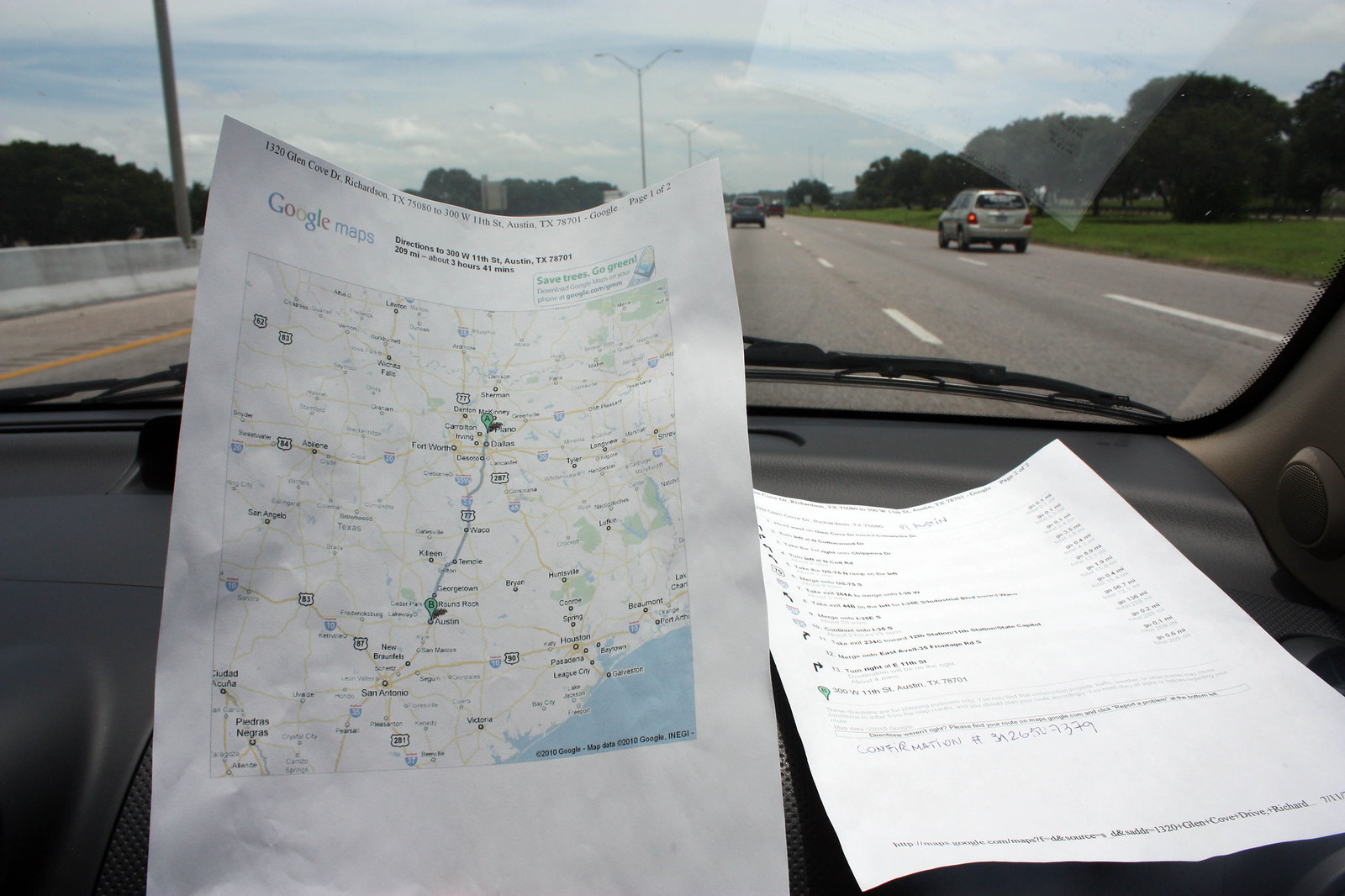The photograph captures the scene from inside a moving vehicle on a highway, focusing on the dashboard, which features a printed map and a set of written directions. The image is taken from the passenger side, providing a view through the windshield that includes a multi-lane highway lined with trees and a grassy area on the right side. The dashboard itself, composed of black plastic, holds two pieces of paper. On the left, an upright piece of paper showcases a Google Maps route, complete with two green pins indicating the starting and ending points connected by a blue line, detailing a trip from Austin to the Dallas-Fort Worth area. This map is presumably being held up, though the hand is not visible. To the right, a flat piece of white paper displays detailed step-by-step written instructions with some handwritten notes at the bottom. Visible at the top of the image are the car’s windshield and windshield wipers, framing a road populated by a few vehicles and set against a clear sky.